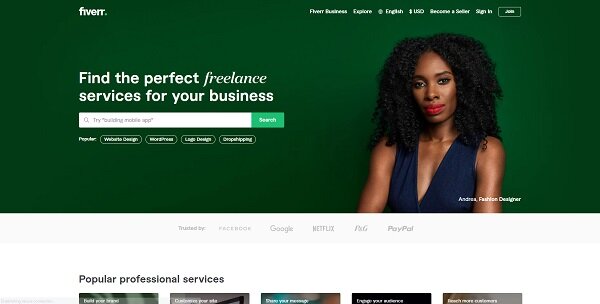The image depicts the homepage of the Fiverr (F-I-V-E-R-R) website. Dominating the top portion of the page is a prominent banner with a dark green background, reminiscent of natural pine tree green. Positioned on the right side of this banner is a photograph of a young Black woman in her 20s or 30s. She is gazing directly at the camera, wearing a navy blue dress and red lipstick, her voluminous curly hair cascading to her shoulders.

To the left of her image, there's a small text identifying her as Andrea, a fashion designer. Adjacent to Andrea’s photo, the main promotional text reads, "Find the perfect freelance services for your business." Beneath this tagline, a search bar is featured, along with suggested popular search terms to aid users in finding relevant freelance services.

At the very top of the page, near the Fiverr logo, there are standard navigation options, including language selection (English), and links to sign in or join the website.

Below the banner, additional information is present in faint text, listing reputable companies that trust Fiverr, such as Peacock, Google, Netflix, P&G, and PayPal. Further down, a subheading reads "Popular Professional Services," accompanied by thumbnails representing various service categories, although these thumbnails are partially cut off in the image.